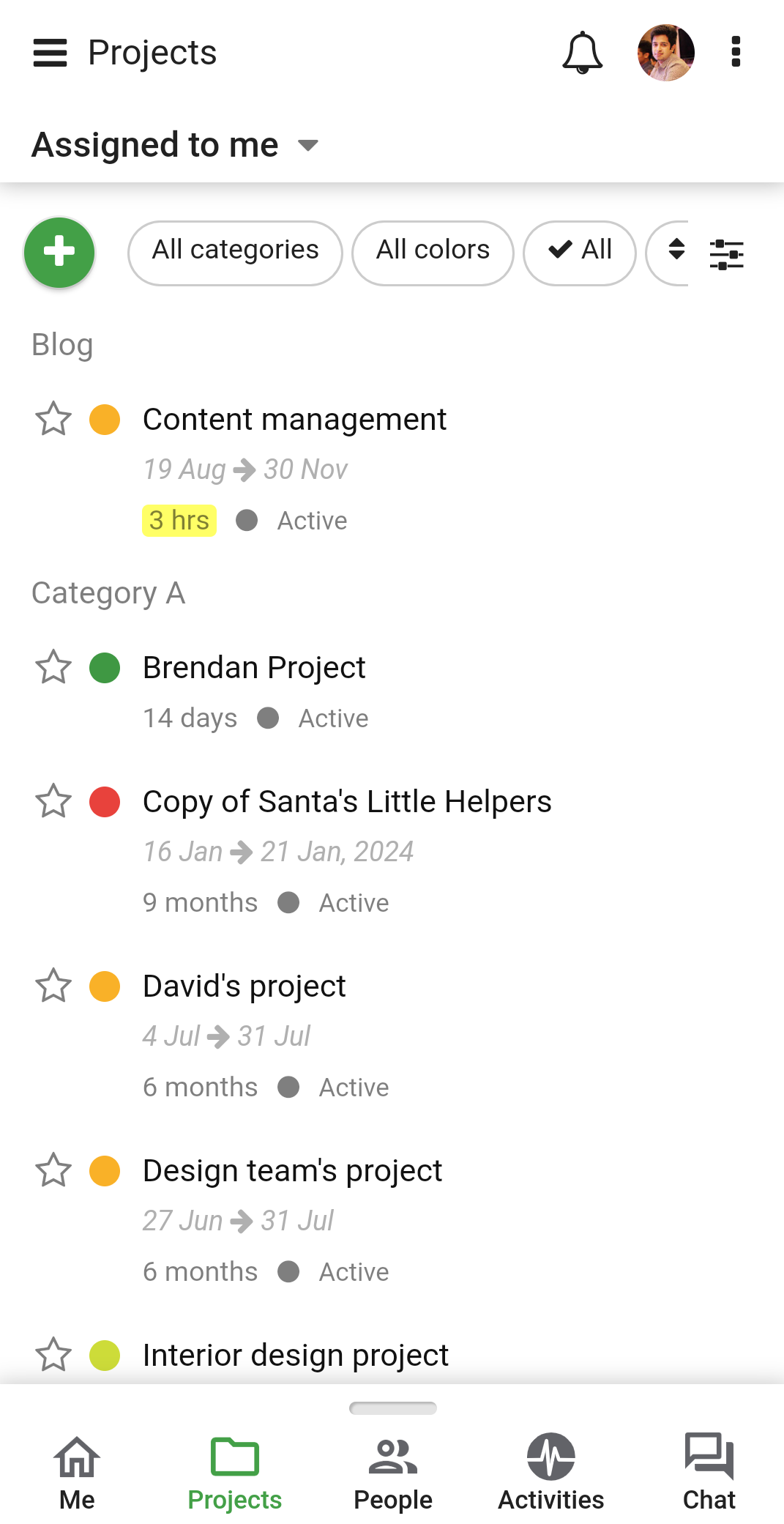A cell phone screenshot displays a project management application with a clean white background. At the top left corner, three horizontal, bolded black lines represent the menu icon. Next to it, the title “Projects” is in black. On the right side, a bell icon, a profile circle, and a vertical ellipsis (three dots stacked) are visible.

Two lines below this, the bolded black text "Assign to Me" appears on the left accompanied by a grey down arrow. A grey horizontal line separates this section from the next.

Below, on the left side, a green circle with a white plus sign is prominent, followed by several filter buttons labeled “All Categories,” “All Colors,” and “All.” The "All" button is checked. Further down, the beginning of another box is visible with an up-and-down arrow icon and an icon depicting three lines with small circles on them.

Approximately two lines down on the left, the word “Blog” is in grey. Two more lines down, a grey outline of a star leads into an orange circle. To the right, the text “Content Management” is present, with “19 AUG” and a right-pointing arrow to “30 NOV” below it. The phrase “three hours,” highlighted in yellow, is followed by a grey dot centered on a line and the grey word “Active.”

Underneath this, the heading “Category A” in grey introduces a list of five projects. Each line starts with a grey outline of a star and a colored dot indicating the project category. The first item has a green dot with the text “Brendan Project.” The second item has a red dot labeled “Copy of Santa's Little Helpers.” The third item has an orange dot for “David's Project,” followed by another orange dot for “Design Team's Project.” The final item features a lime green dot for “Interior Design Project.”

At the very bottom, navigation buttons are labeled “Me” (home button), “Projects,” “People,” “Activities,” and “Chat.”